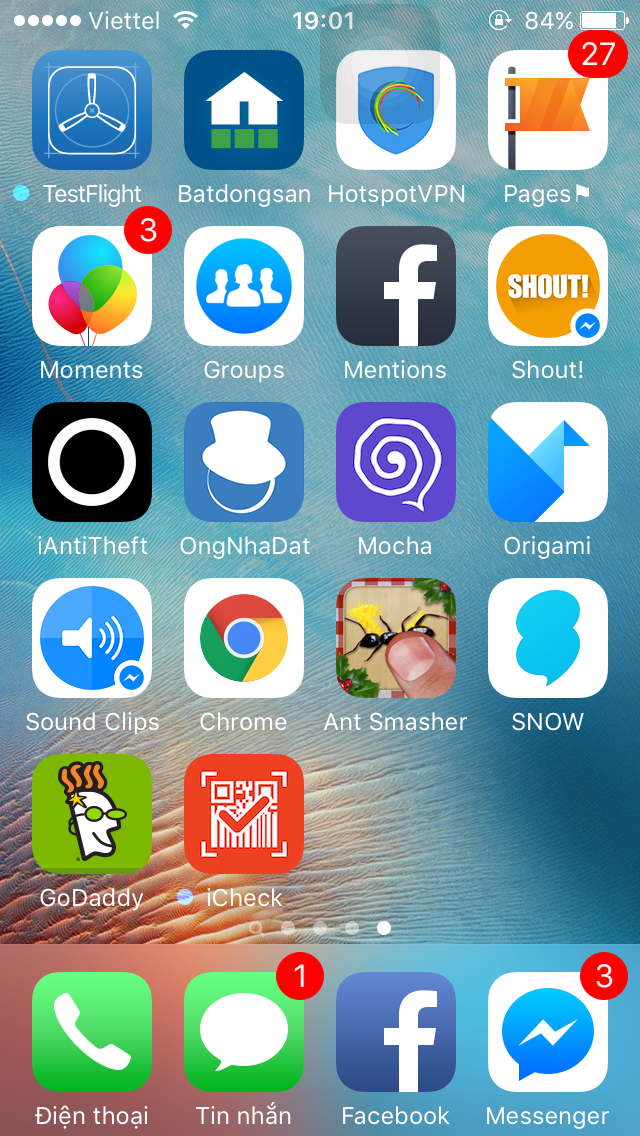The image displays a smartphone screen filled with a variety of apps. At the top, the network carrier "Viettel" is prominently displayed in white letters, alongside the time "19:01" and a battery icon indicating an 84% charge. Below the battery icon is an app labeled "Pages," which has a red notification badge with the number 27 in white. 

The first row of apps includes "TestFlight," "BatDogSun," "Hotspot VPN," and "Pages." The second row features "Moments," "Groups," "Mentions," and "Shout." The third row displays "AntiTheft," "Antna," "Dot," "Loka," and "Origami." The fourth row consists of "SoundClips," "Chrome," "AntSmasher," and "Snow." The final row shows "GoDaddy" and "iCheck."

At the bottom of the screen are icons for essential functions: Phone, Messages, Facebook, and Messenger. The Messages app shows a notification badge with a "1" in the upper right corner, while Messenger has a "3" in the same position.

The app icons are set against a blue background with brown accenting the lower right and left corners.